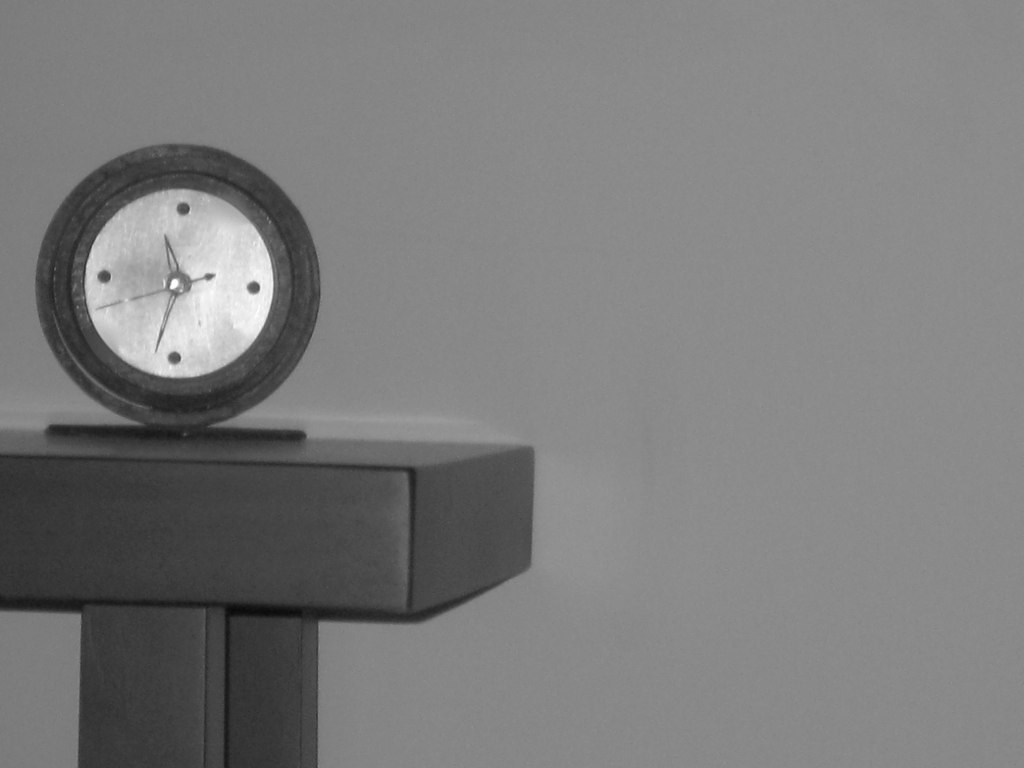The image is a piece of digital art that appears very realistic. It depicts a black and white scene with a medium gray background. Positioned prominently on the left side is a round clock resting on a dark tabletop. The clock features a frame that resembles wood, creating a striking contrast with its lighter, shiny, silver face. Instead of numbers, the clock has four large dots marking the 12, 3, 6, and 9 o'clock positions. It has three hands: a minute hand, an hour hand, and a second hand. The time displayed is approximately 11:32. The tabletop has a T-shaped design, and the overall color scheme of the image is various shades of gray, lending it a monochromatic aesthetic.